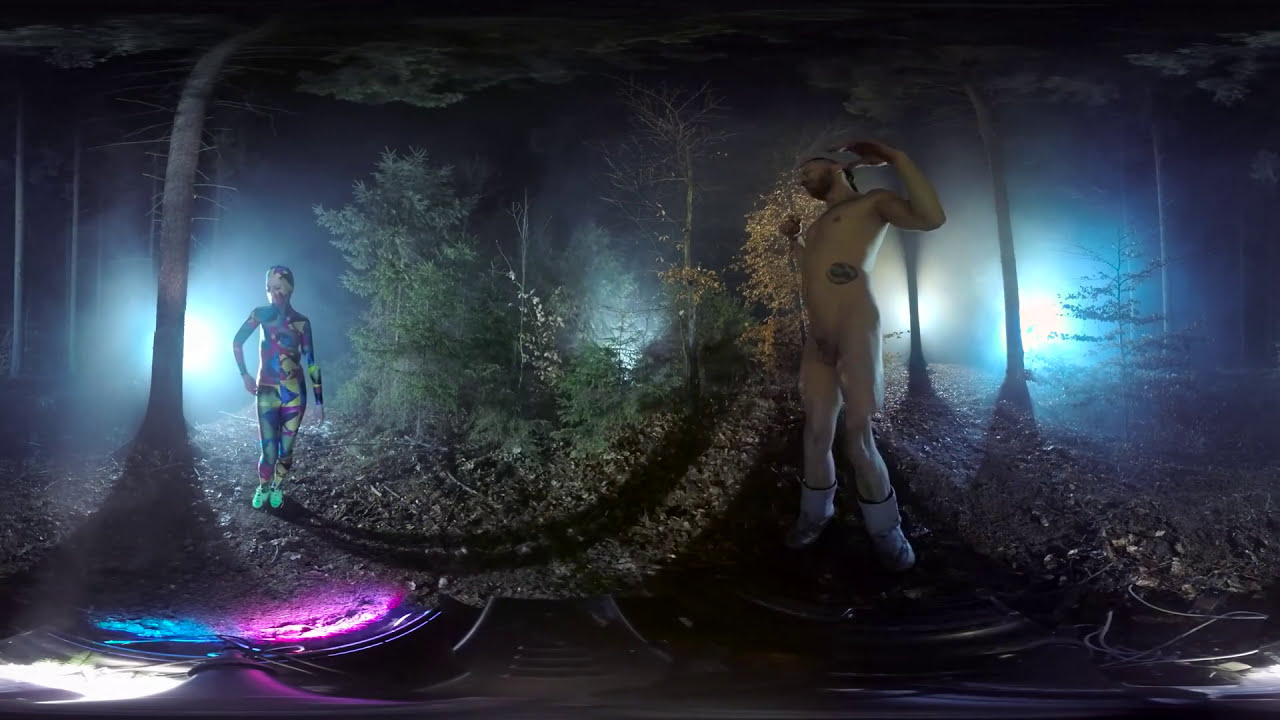The image depicts a dark, forested area that seems to come straight out of a video game. The scene is set at night, with a dense arrangement of trees, some adorned with leaves while others stand bare. The ground is covered with soil, scattered leaves, and twigs, adding to the natural feel of the wooded environment.

On the left side of the image is a female-shaped character, striking a dynamic pose with one hand on her hip and the other hanging down by her side. This character is peculiar, covered in an abstract pattern featuring shades of blue, gold, and purple, and is adorned with greenish white tennis shoes. A notable feature is what appears to be a creature-like tail extending from this character toward the right side of the image.

To the right stands a nearly naked man, identifiable by a tattoo on his left abdomen. He is only wearing boots and has his arms raised above his head, elbows slightly bent, and possibly wearing a blindfold. His stance is open, adding to the surreal feel of the scene.

The background is illuminated by intense, globe-like spotlights in hues of blue and yellow, which cast dramatic shadows of the trees onto the ground. Additional colorful lights in pink, purple, and blue create a misty haze, particularly noticeable towards the top and bottom left corners of the image. Near the bottom of the picture, the abstract design continues with splashes of purple, blue, and black, possibly hinting at the hood of a car or another undefined object.

The combination of atmospheric night lighting and the unique, vividly colored characters gives the image a mystical, almost otherworldly quality, immersing the viewer in a digital fantasy forest.